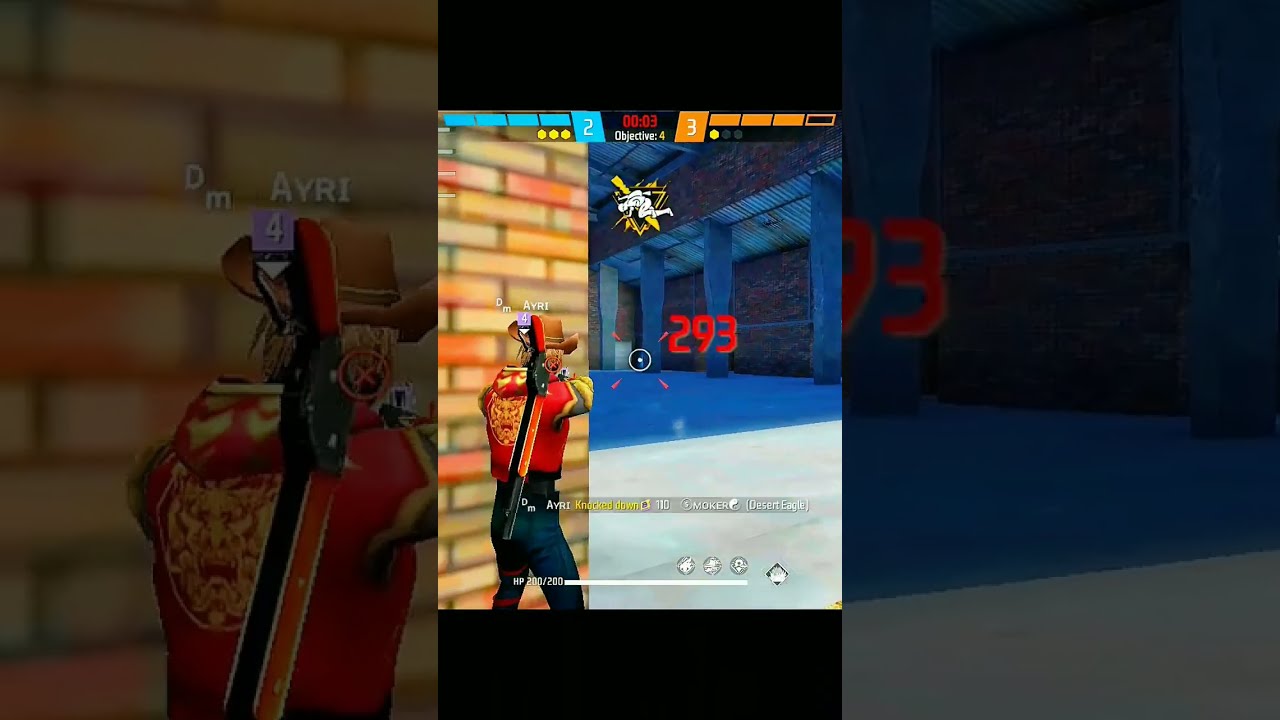The image is from a video game displayed on a tablet, resulting in the left and right sides being zoomed-in, blurred extensions of the main scene at the center. The focal point is a third-person view of a cowboy character named A-Y-R-I, who is taking cover against a multicolored brick wall featuring shades of yellow, red, brown, and orange. The character, A-Y-R-I, is dressed in a red vest emblazoned with a yellow dragon or Viking symbol on the back and sports a brown cowboy hat and black pants or blue jeans. Slung across his back is a shotgun or a sword-shotgun hybrid weapon. A-Y-R-I's arms are raised, potentially holding a gun that seems clipped into the adjacent wall.

To the right of the character, there is an aiming reticle, a circle with a dot in the center, and a "293" in red, possibly indicating damage dealt. Above this, a score and status bar show the time as "0:03" seconds left, with "Objective: 4". The scoreboard indicates the blue team with a score of 2 and three small circles, while the orange team has a score of 3 and one small circle. Additionally, a lightning-struck falling character icon beneath the timer could signify a downed player or a skill effect.